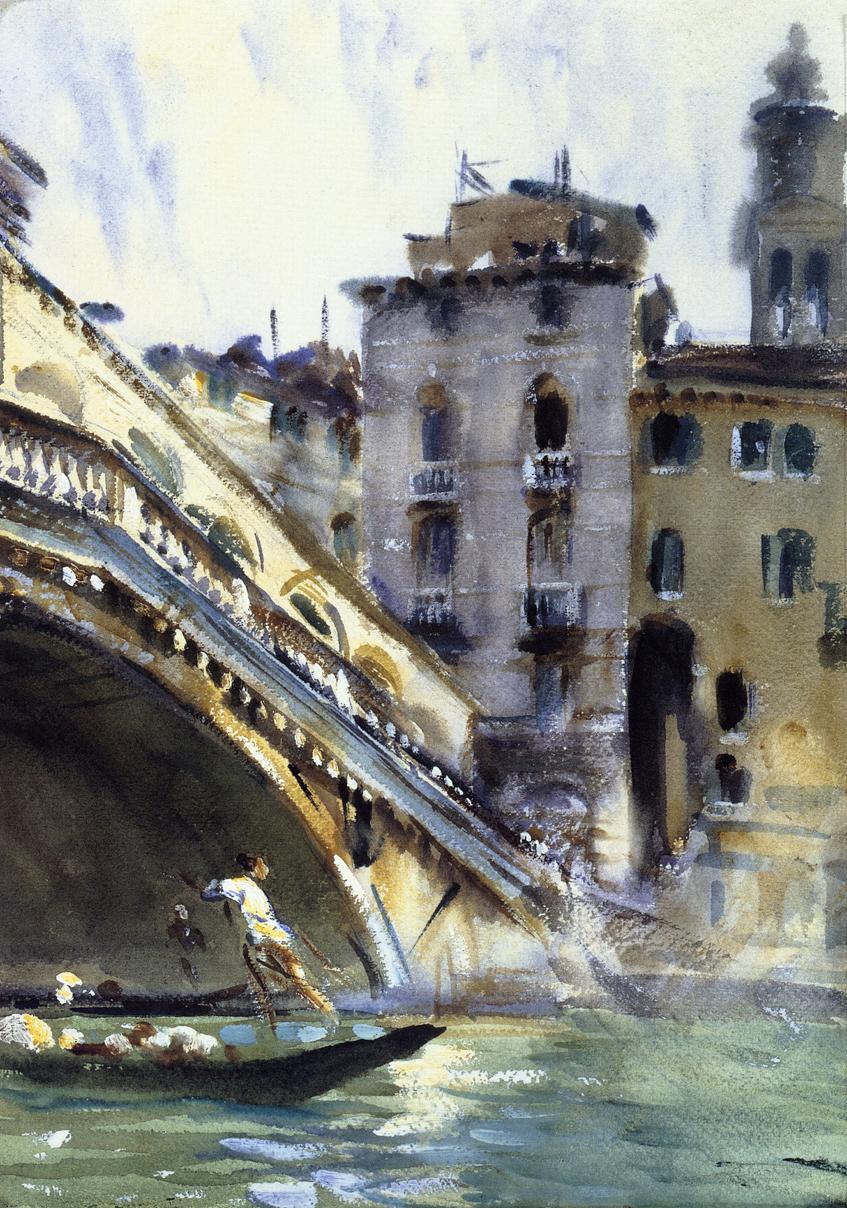This detailed painting depicts a serene Venetian scene with a gondola gliding beneath a partially visible bridge over a greenish river. In the foreground, a gondola operator, standing in white attire with dark hair, navigates the vessel. Behind him, some indistinct packages are visible. The bridge itself is an amalgam of brown, cream, and light blue hues. To the right of the painting are numerous multi-storied buildings, some gray, beige, yellow, and light pink, each adorned with several windows and one featuring a prominent tower on its roof. In the distance, another gondola with a standing figure can be faintly observed, adding depth to the scene. The sky above is a soft blend of blue and white, sprinkled with clouds, suggesting a clear, sunny day. The painting captures the timeless essence of Venice with meticulous detail and a hint of nostalgic blur.